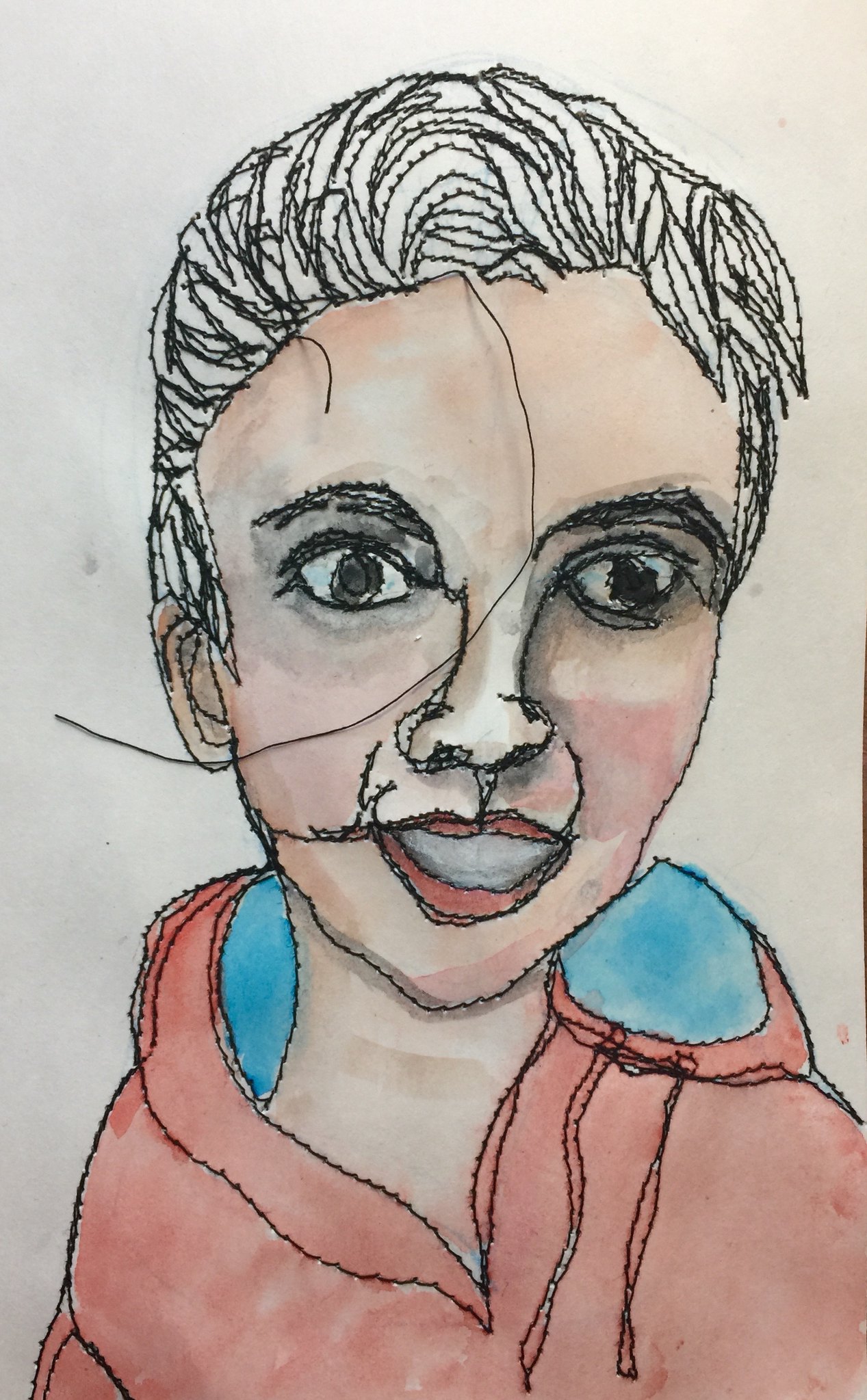This vertically oriented piece of art is a meticulously detailed portrait of an individual wearing a light red or pink jacket accented with a blue collar. The outer edge of the image, along with the intricate details, appears to be stitched with black thread, adding a distinct textured effect. The subject's hair is intricately detailed with long and short threads extending from the hairline onto the forehead, and a long, wispy thread gracefully trails over the nose towards the left of the face. The facial features are vividly rendered, showcasing bright, black-colored eyes, wide eyebrows, a short, stout nose, and slightly parted lips. Both the face and the coat are subtly shaded with a wash effect, creating a lighter tint that highlights the contours of the face, neck, and jacket. The background serves as a contrasting backdrop with its off-white, grayish hue.